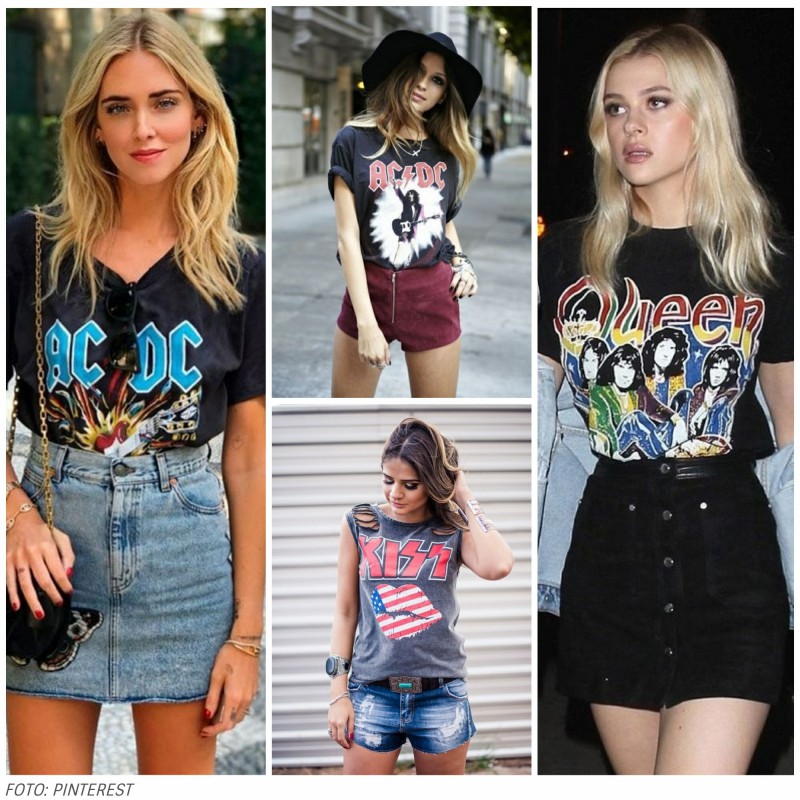The image is a collage of four photographs featuring young women, each modeling rock-and-roll band t-shirts, all likely from the 70s and 80s era. 

On the left, a blonde woman is dressed in a black ACDC v-neck t-shirt featuring aqua-blue lettering and a red guitar with explosive graphics. She complements this with a denim mini skirt, a black handbag with a gold strap, sunglasses hanging from her shirt, and accessories including bracelets, nail polish, and a band on her finger. 

In the center, the top image displays a woman with light brown hair wearing a black ACDC t-shirt with red lettering and an image of a guitarist. She pairs this with maroon shorts and a black cowboy hat. Below her, another woman has darker brown hair and dons a gray KISS t-shirt with red lettering and an American flag design. She is also clad in denim short shorts with a large silver-buckled belt, red nail polish, and a sizable watch on her right wrist.

The woman on the right has blonde hair and is sporting a black t-shirt with the word "Queen" emblazoned on it, along with a graphic of the band members. She pairs this with a black denim mini skirt, adding a modern touch to her classic rock look.

Overall, the collage not only showcases different rock band t-shirts but also highlights a variety of personal styles and accessories, merging vintage themes with contemporary trends.